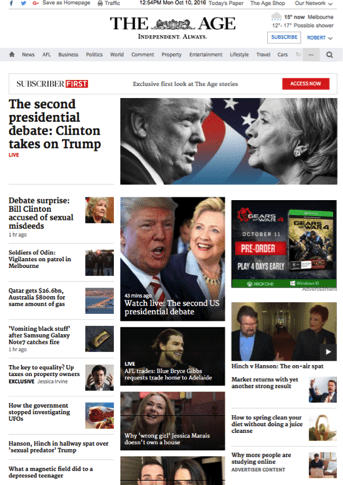This is a detailed screenshot of a news website titled "The Age, Independent Always." The webpage is captured at 12:54 p.m. on Monday, October 10th, 2016. Prominently, the main headline in large font reads, "The Second Presidential Debate: Clinton Takes on Trump," accompanied by a striking black-and-white image of Donald Trump and Hillary Clinton facing off, their side profiles highlighted against a vibrant red, white, and blue backdrop resembling the American flag.

On the left-hand side, a vertical menu showcases various headlines alongside smaller thumbnail images. These headlines include, "Debate Surprise," "Bill Clinton Accused of Sexual Misdeeds," "Soldiers of Odin: Vigilantes on Patrol in Melbourne," "Qatar Gets $26.6 Billion, Australia $800 Million for Same Amount of Gas," "Vomiting Black Stuff After Samsung Galaxy Note Catches Fire," and "The Key to Equality: Up Taxes on Property Owners."

Meanwhile, the right-hand side features a series of larger thumbnail images that correspond to different stories, with text overlaid on each image, providing a visual summary of the news articles. This layout presents a comprehensive and dynamic overview of the day's major news events and trending stories, encapsulated within an informative and visually engaging online newspaper format.